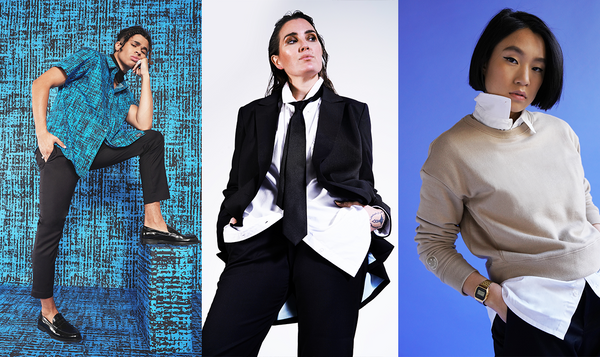The image consists of three fashion photographs, each featuring a model posed against distinct backdrops, showcasing different styles but unified in framing and composition.

On the far left, a young Caucasian man poses against a turquoise background that matches his turquoise shirt with black markings. He is dressed in black trousers and black slip-on shoes. His dark hair falls to his shoulders as he rests one foot on a platform, with his left elbow placed on his raised knee, his hand supporting his chin, and his right hand in his pocket.

In the center, a Caucasian woman stands against a white background, exuding a business-like appearance. She wears a dark-colored suit paired with a white shirt and a matching dark tie. Her dark hair contrasts against her light makeup. The white shirt is slightly untucked, giving a casual touch to her otherwise formal attire. She also sports black trousers, completing her authoritative look.

On the right, an Asian woman stands against a blue background. She has short dark hair, styled casually to one side. She wears a white shirt with an oversized collar that peeks prominently from under her brown-colored sweatshirt. Black trousers and a bronze-colored wristwatch add to her ensemble, giving off a stylish and laid-back vibe. Her hands are casually tucked into her pockets.